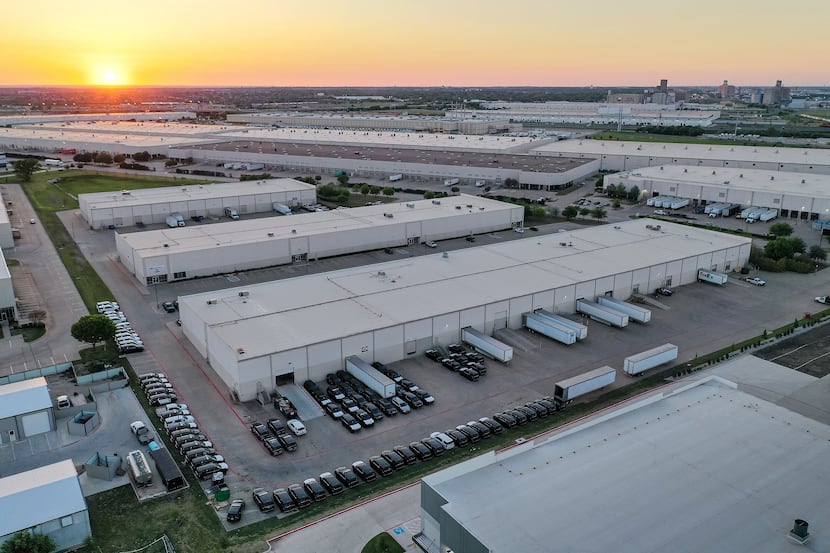An aerial photograph captures a sprawling industrial landscape dominated by numerous one-story, white shipping warehouses with flat roofs. These buildings, reminiscent of factories, extend across the entire field of view, with at least ten prominently visible. The foreground showcases a warehouse with several open doors, in front of which long semi-trailers are parked. Surrounding this building are rows of parked cars. Adjacent to it, another identical warehouse is visible but lacks the trailers and cars of its neighbor, while a third, shorter warehouse in the triangularly narrowing plot has a few trailers and cars around it. The flat roofs of these warehouses are dotted with protrusions likely for heating and air conditioning units. Along the horizon, spanning the entire width of the photo, a sunset casts a yellowish-gold hue on the left side of the sky, transitioning to gray, yellow, and pink towards the right. The industrial scene is complemented by distant buildings in the upper right section of the photo, creating an overall flat terrain devoid of mountains or hills. The presence of numerous black cars and white storage containers scattered across the area further emphasizes the extensive use of the space.